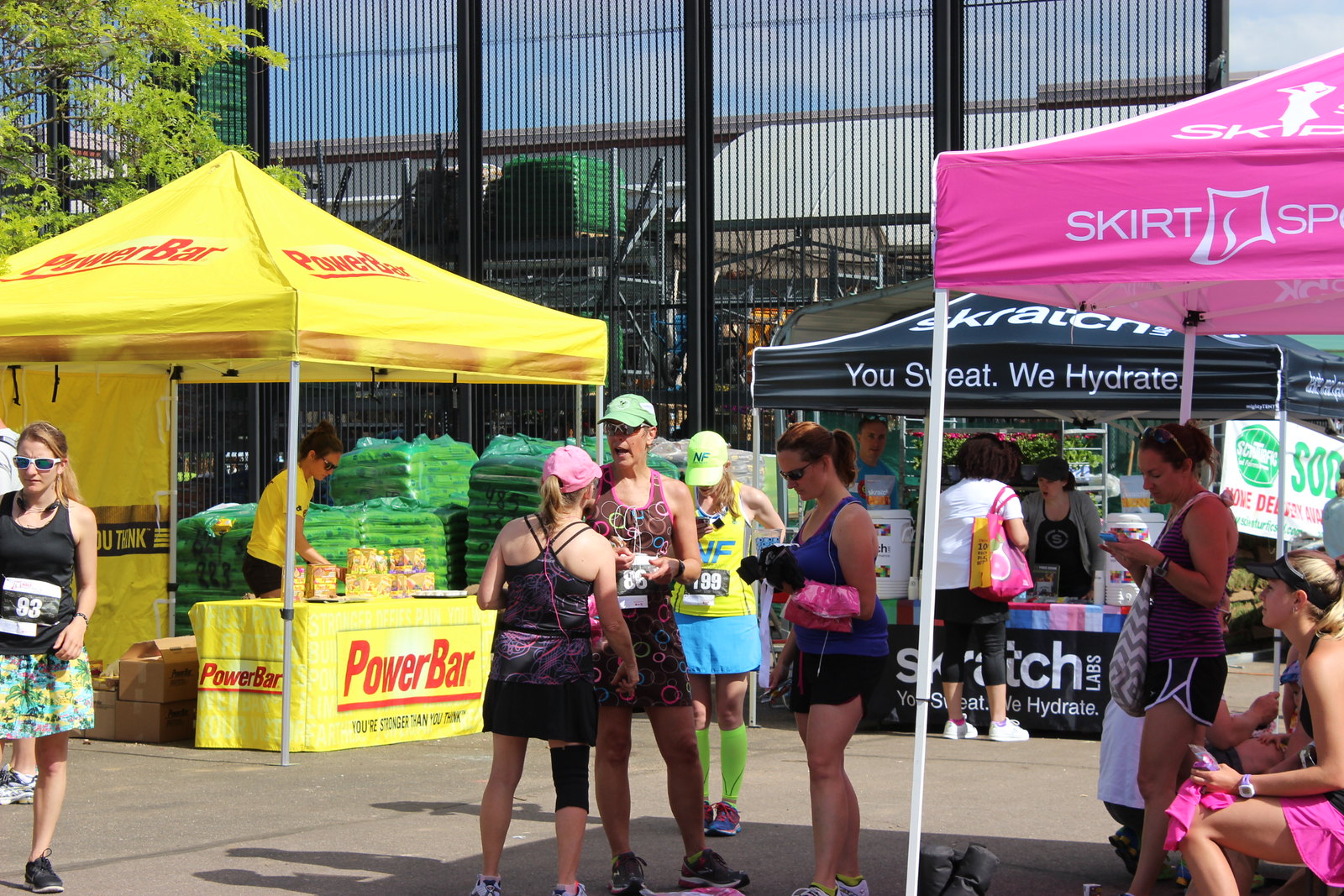The photograph, taken outdoors during the day—likely in a parking lot outside a garden section of a Lowe's or Home Depot—captures a bustling scene from a benefit road race. Numerous participants, both men and women, are clad in athletic attire, with bib numbers pinned to their chests. Prominent among the structures is a yellow tent marked with the "Power Bar" logo in red, staffed by a woman in a yellow shirt manning a table stocked with power bars. Nearby, a black tent displaying the slogan "Scratch, you sweat, we hydrate" hosts individuals sampling hydration products, including a woman in a white shirt, black pants, and white sneakers. To the right of the image stands a pink tent branded “Skirt SP,” under which a blonde woman in a pink skirt and visor sits alongside another woman in a black tank top and shorts engrossed in her phone. Between the yellow and pink tents, a man in a green baseball shirt and tank top with the bib number 86 converses with a woman wearing a black tank top, skirt, knee brace, and pink cap. Nearby, a woman in a green floral print skirt, black tank top, and bib number 83 stands. In the background, metal fencing and pallets of fertilizer in green packaging delineate the setting, suggesting the garden section of a large retail store.